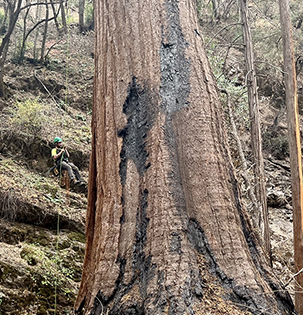The almost square photograph captures a towering giant tree dominating two-thirds to three-fourths of the frame, dwarfing the surrounding smaller forest that appears to rise steeply behind it, as if on a mountainside. A tiny figure, a man, can be seen rappelling or climbing the tree with the aid of a green rope extending from the base to beyond the top of the image. His green helmet and yellow shirt, paired with grey pants, make him slightly more noticeable against the vast brown and black hues of the tree's bark, which is heavily scarred and showing signs of age or damage. The immense scale of the tree is emphasized by how small the man appears—he is nearly unnoticeable and probably covers just a tenth of the tree's width. The surrounding forest, filled with regular-sized trees and thick shrubbery, enhances the grandeur and apparent age of the giant, possibly a red oak, in the foreground.